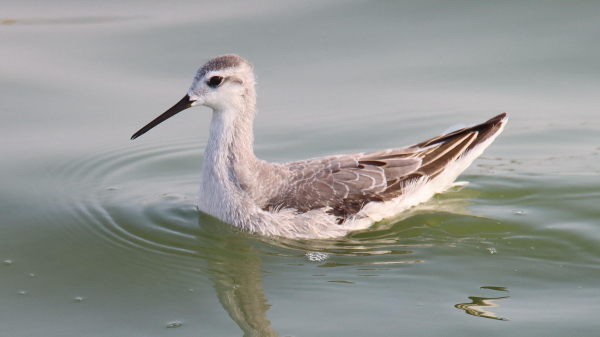This high-definition nature photograph captures a tranquil scene of a small pond or lake. The water, primarily light blue with a greenish tint, occupies most of the rectangular frame, which is wider than it is tall. The serene water surface shows gentle ripples and a few bubbles, punctuated by the reflection of a bird sailing gracefully. 

The bird in the image has a distinctive long, slim black beak and is seen in profile. Its body is mostly white, with a grey top of the head and grey feathers that transition to black along the back. The tail feathers are a striking chocolate brown. Although the bird's feet are submerged, its peaceful demeanor and the detailed reflection in the water add to the photograph's calming atmosphere. Overall, the image presents a serene and picturesque glimpse of the bird navigating the calm, slightly greenish waters.